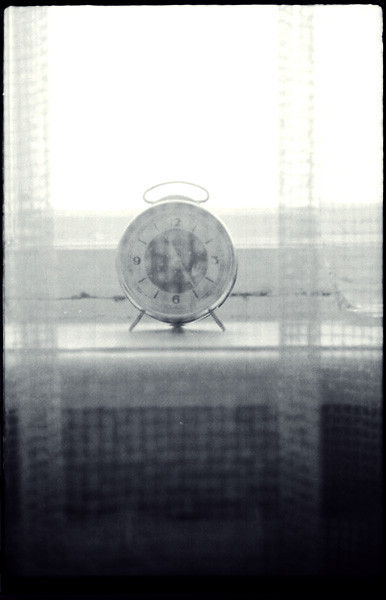A small, round alarm clock with a chrome metal frame is showcased in the image. The clock features an oblong handle at the top and rests on a short stem, flanked by two stabilizing legs. Its face is a combination of dark and white colors with black numbers and white hour and minute hands. Positioned on a white windowsill, the clock is bathed in light streaming through a white, translucent curtain. The curtain partially obscures the bright scene outside, adding a soft, diffused glow to the entire setup.